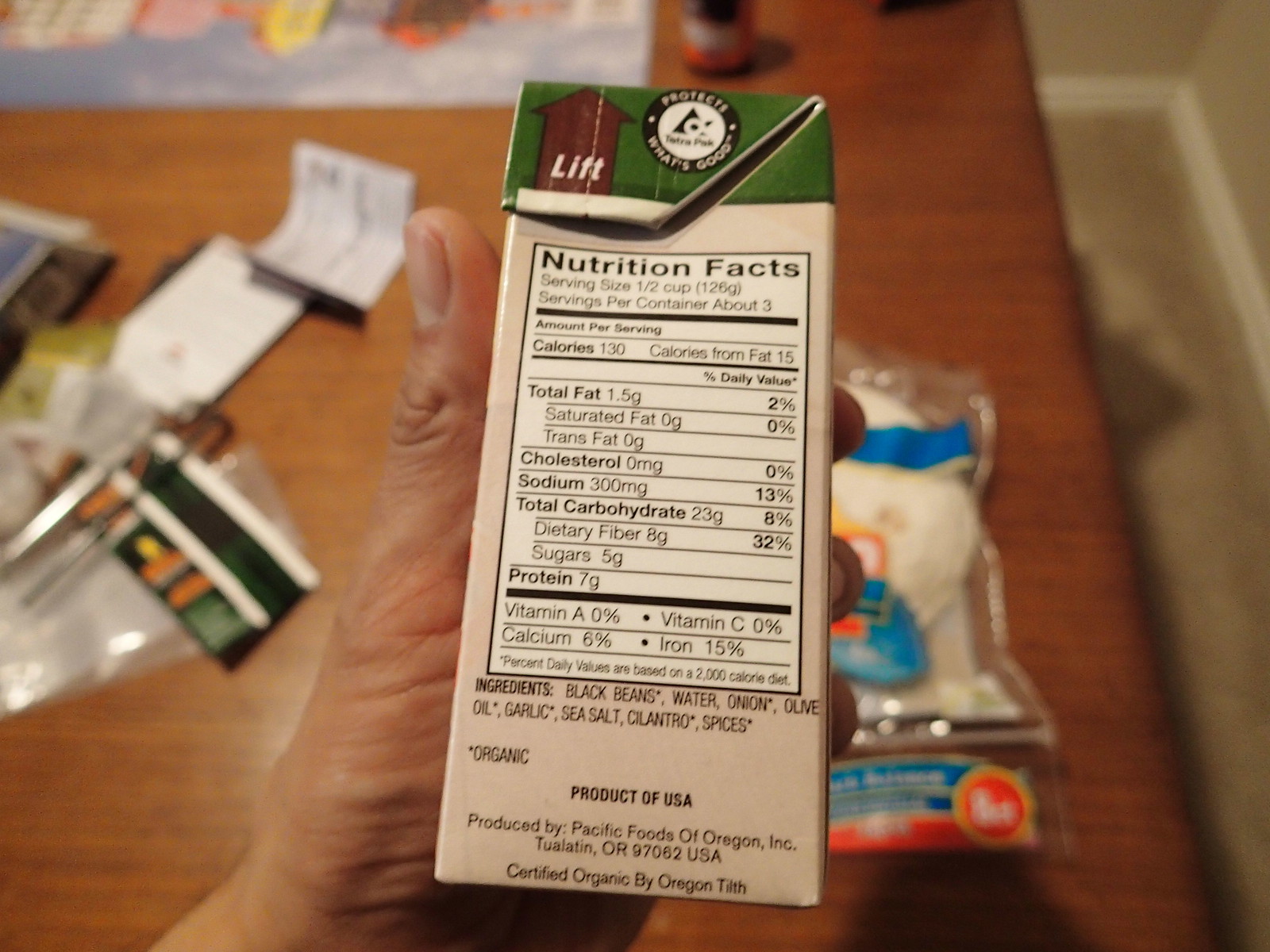The image depicts a carton containing an organic food item. The carton features a tab clearly labeled "LIFT" to facilitate opening. Displayed on the side of the carton are detailed nutrition facts. The serving size is listed as half a cup, with the carton containing approximately three servings. Each serving provides 130 calories. The total fat content is 1.5 grams, contributing to 2% of the daily recommended value, with no saturated or trans fats present. The cholesterol level is also zero. The sodium content is 300 mg, accounting for 13% of the daily value. In terms of carbohydrates, the total is 23 grams, which is 8% of the daily value. The dietary fiber content is notably high at 8 grams, representing 32% of the daily value, and there are 5 grams of sugars. The list of ingredients includes black beans, water, onion, olive oil, garlic, sea salt, cilantro, and spices, highlighting the product's wholesome and organic nature.